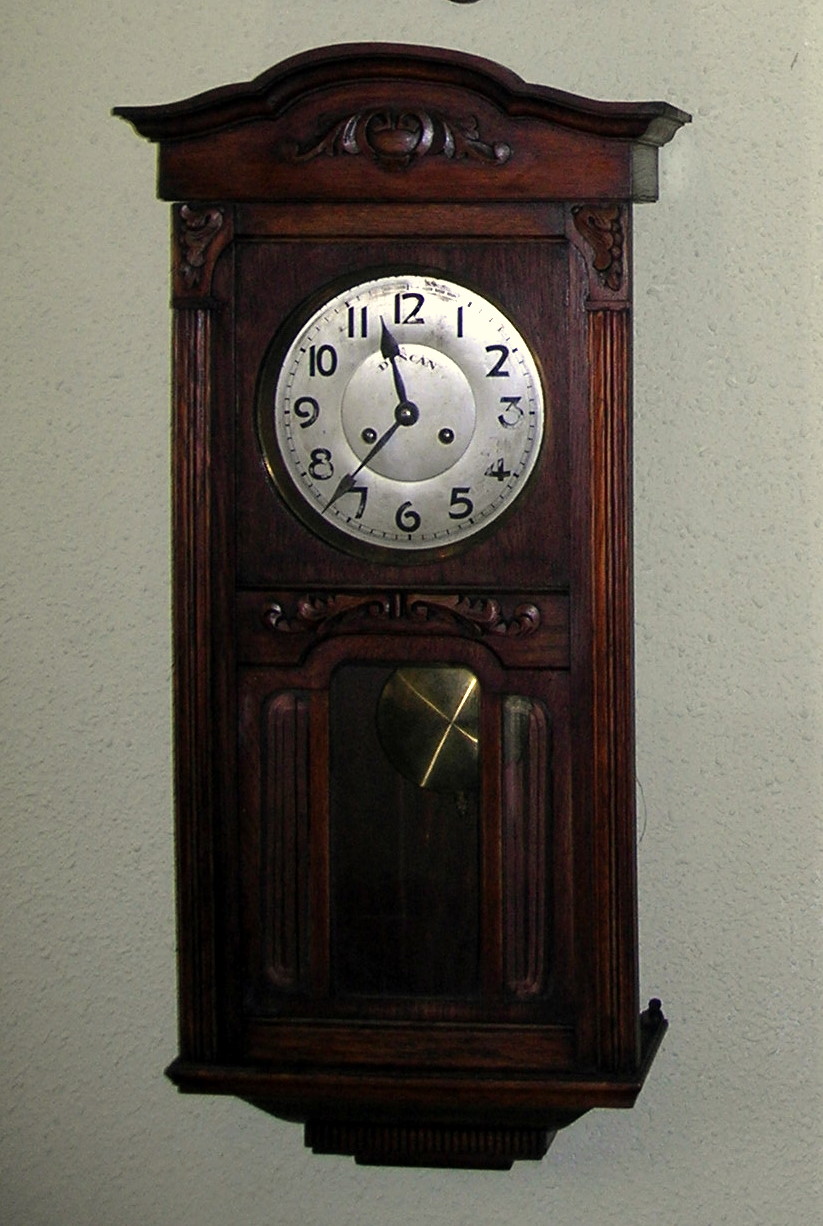This photograph captures a vintage wall clock with classic grandfather clock aesthetics. The clock, crafted from dark mahogany wood with a burgundy undertone, showcases intricate woodwork, including 3D geometric shapes and vertical lines around the border. The centerpiece, a large, slightly worn silver face inscribed with "Duncan," features numerals from 1 to 12, with notable wear on the numbers 3 and 4. Time is marked at 11:37, with the hour hand between 11 and 12, and the minute hand slightly past 7. The clock boasts a charming pendulum visible through a small door at the bottom, adding to its antiquated appeal. The background plastered stucco wall further enhances the vintage charm of the piece.